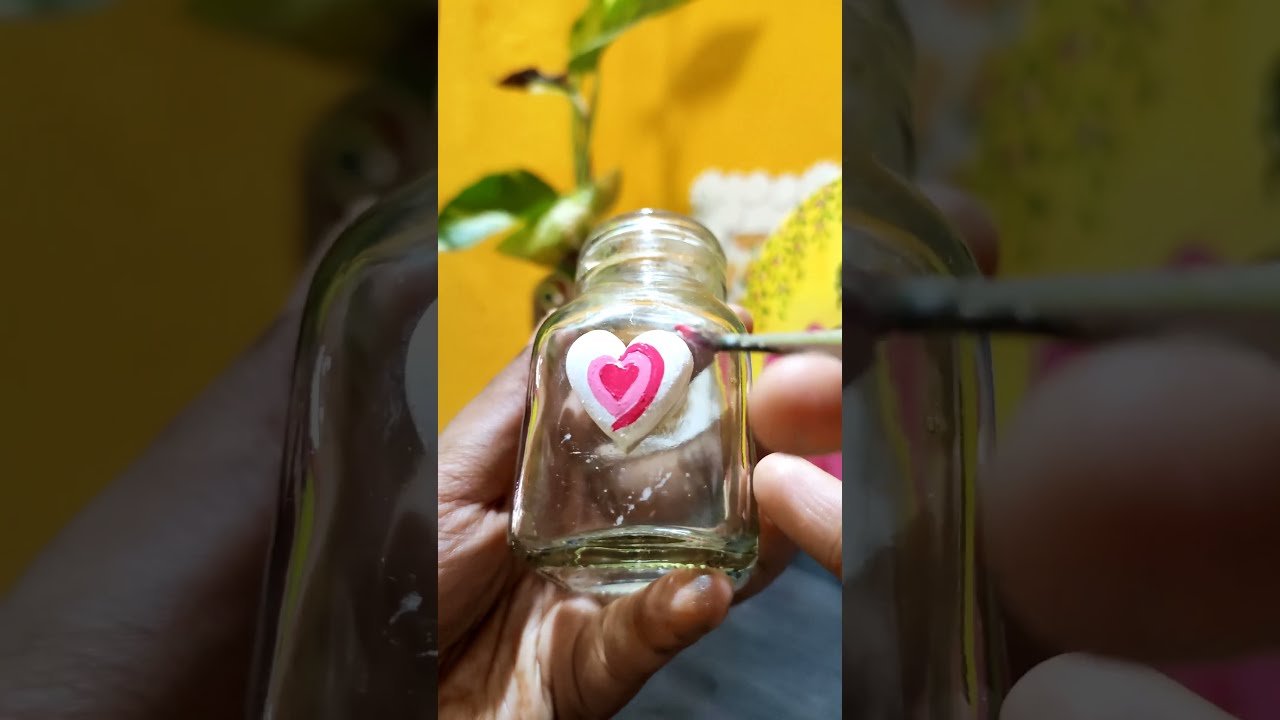This image is a detailed, rectangular portrait orientation photograph centered on a person's hand holding a small, transparent glass jar, resembling a salt and pepper shaker or a tiny mason jar. The background features a yellow wall with a green plant extending upward, slightly shadowed on the left and right sides of the image. The jar, open at the top, serves as a canvas for a multi-layered heart painting. The person's right hand is seen applying paint with a brush to the jar. The painting features a large white heart bordered with a partially painted pink outline, followed by a smaller pink heart, and a tiny red heart nestled at the center. The details of the layered hearts have a sequence of white, pink, and red colors. The zoomed-in and darker side portions of the image emphasize the central elements, guiding the viewer's focus to the jar and the painting process.